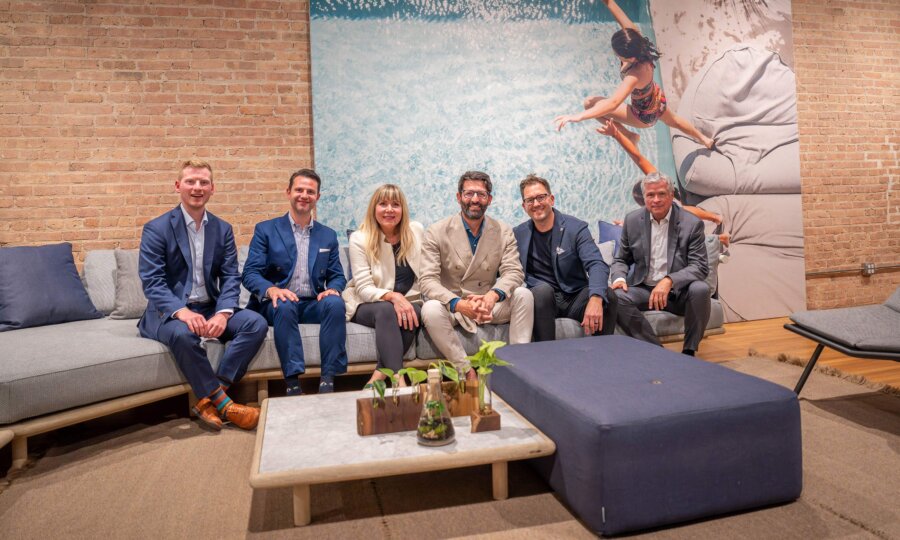This photograph features a group of six people, five men and one woman, all dressed in business attire and seated on a large gray sectional sofa. The woman is seated third from the left. The men include three in blue suits, one in a beige suit, and an older gentleman in a gray suit with white hair. Directly in front of them is a low white marble coffee table with wooden legs, adorned with potted pothos plants and glass beakers containing seedlings and plant grafts. To the right of the coffee table sits a substantial navy blue ottoman. Further to the right, a sliver of a gray-cushioned chair is visible. The group is positioned on a tan-colored fabric rug, which covers most of the room's floor, save for a glimpse of wood flooring on the right side. They sit in front of an exposed red brick wall that features an extremely large photograph of two children jumping into a pool from an aerial view. All members of the group are smiling, posing harmoniously for the picture.